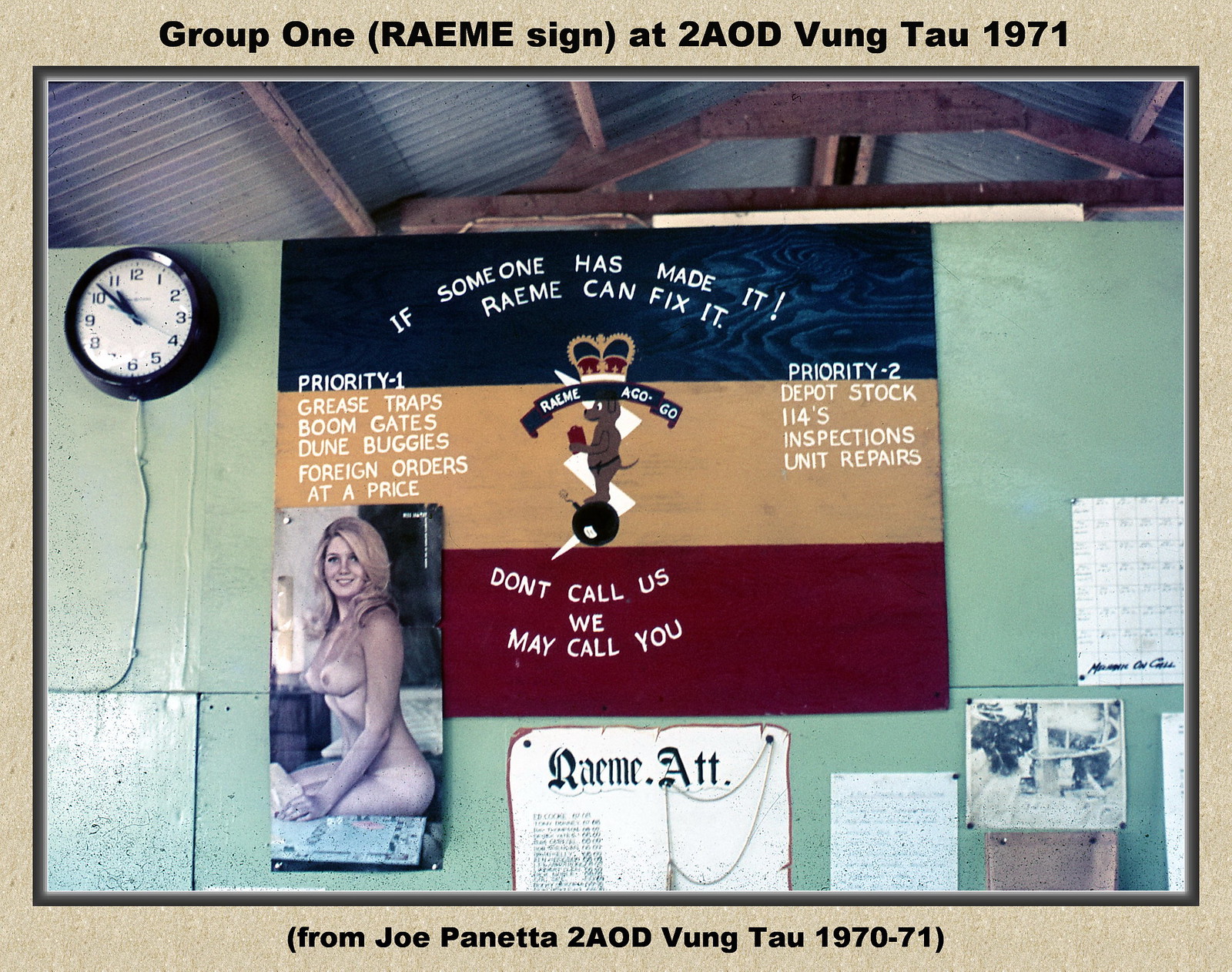This horizontally aligned rectangular picture depicts the interior of a pavilion with a sheet metal roof supported by wooden beams. The main feature is a decorated grayish-brown wall adorned with various items. Prominently displayed in the center is a large, striped banner with sections of navy blue, brown, and red. The banner reads, "If someone has made it, R-A-E-M-E can fix it" in white text, with an image of an animal wearing a crown below. Below this, against the red background, it says, "Don't call us, we may call you." To the left of the banner is a black-rimmed wall clock showing the time as 10:53. Near the banner, there is a poster of a naked woman with long blonde hair, posed on her knees. Above these elements, the text reads, "Group 1 (R-A-E-M-E sign) at 2 AOD Vong Thao, TAU 1971." Further below, more text in black letters mentions, "From Joe Panetta to AOD Vong Thao 1970-71." The wall is further decorated with smaller, unreadable signs and a calendar positioned to the right, making it appear as though the wall serves as a bulletin board of sorts.